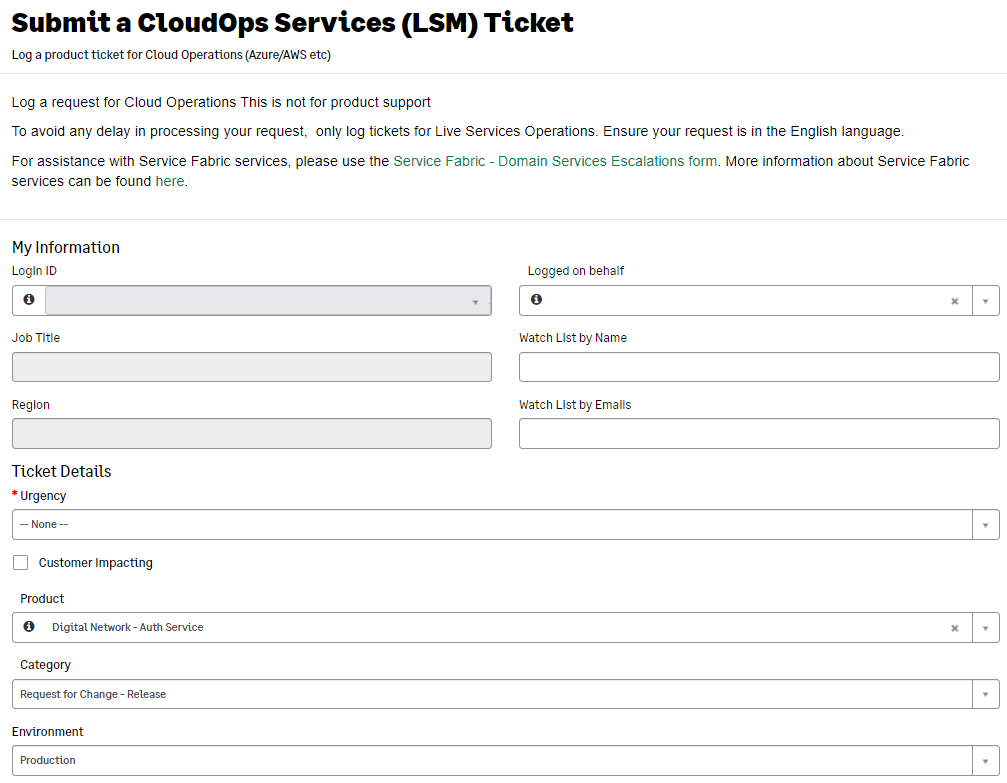The screenshot displays a page from a website with a clean, white background. Positioned at the top left, large, bold black text reads "Submit a CloudOps Service (LSM ticket)." Directly below, in smaller black text, it states, "Log a product ticket for cloud operations (Azure/AWS, etc.)." A thin, light gray horizontal separator line follows.

Underneath the line, there are four lines of small black text:
1. "Log a request for cloud operations. This is not for product support" (without a period).
2. "To avoid any delay in processing your request, only log tickets for live services operations. Ensure that your request is in the English language."
3. "For assistance with service fabric services, please use the," highlighted in green, "service fabric - domain services escalations form."
4. "More information about service fabric services can be found," also highlighted in green, "here."

Another thin, light gray horizontal line appears below these instructions.

In the top left of the subsequent section, bold, dark gray text reads "My Information." Below this header, there are text entry boxes with medium gray outlines and titles positioned to the upper left in small black text. The first entry box is labeled "Login ID." This box includes a light gray drop-down menu with a medium gray triangle pointing down on the right. Additionally, on its left side, there is a white square featuring a white eye icon encircled by a black outline.